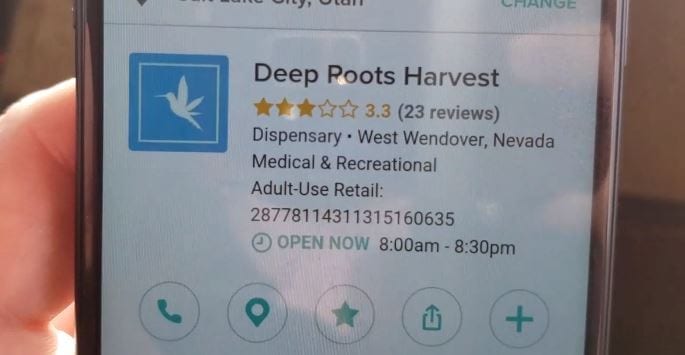In this detailed close-up color photograph, the central focus is a vertically-held smartphone being displayed by a hand positioned to the left. The screen prominently features a listing for Deep Roots Harvest Dispensary, located in West Wendover, Nevada. The dispensary caters to both medical and recreational adult use and boasts a rating of 3.3 stars from 23 reviews. Below this, the text indicates the dispensary's operating hours from 8:00 a.m. to 8:30 p.m. The display includes a string of numbers, likely the contact details, along with various icons such as phone, map, favorite, forward, and add. The listing also features the dispensary's logo—a blue square with a white hummingbird. The color palette in the image includes peach, brown, blue, white, green, black, deep yellow, orange, light blue, and turquoise. The overall setting seems to emphasize that the phone is being held up to show the screen information.